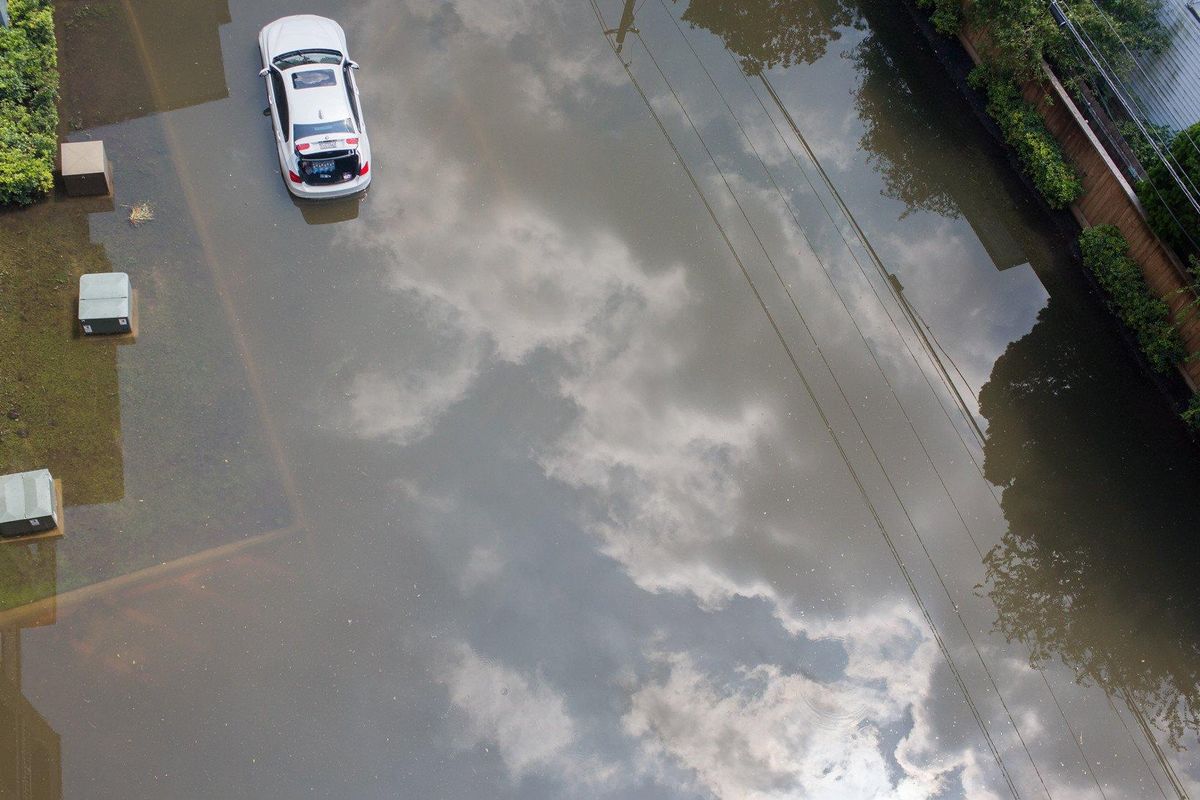An aerial view reveals a town submerged in murky brown floodwater, which extends over various properties and green spaces. The floodwater partially covers the vibrant green grass in a garden, making the submerged foliage visible beneath the surface. A white saloon car, with its boot open, is parked amidst the inundation, though it’s unclear if anyone is inside. The bright, sunny day features white clouds that reflect on the water’s surface, enhancing the scene’s surreal and tranquil atmosphere. Alongside the road, several lush green trees stand tall, unaffected by the floodwaters. An electric pole, reflected in the water, adds to the structural elements visible in the image. No human presence or animals are discernible in this flooded landscape, emphasizing the stillness and quiet of the scene.